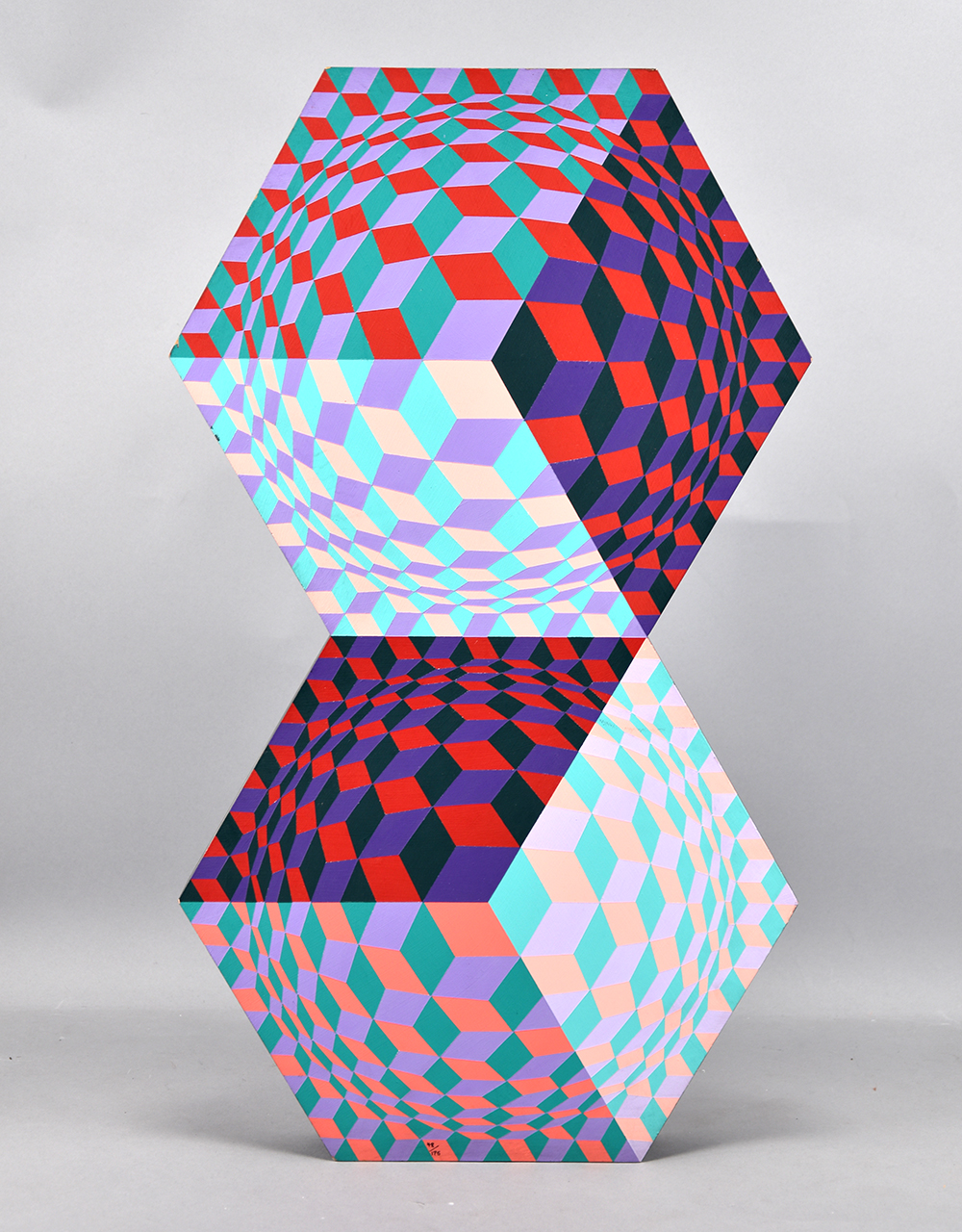This image features two large, geometrically shaped cubes, each approximately five feet per side, stacked on top of one another at a tilted angle, with the backdrop being a plain white surface. The cubes are aligned such that the top cube appears to be balanced precariously on the sharp edge of the bottom cube, creating an abstract and visually intriguing composition akin to a modern art installation. The design on each cube's face resembles a Rubik's Cube, with vibrant, contrasting colors. The top cube showcases a dynamic blend of colors, including reddish-black transitioning into green with hints of red, complemented by patches of purple and a striking hot blue. The bottom cube features a similar palette but with a distinct arrangement: dark reddish-purple at the top, fading into lighter shades of red and purple, alongside green and a yellowish hue on its sides. This intricate pattern of colors and the cubes' tilted, almost cascading orientation gives the image a unique, abstract feel, blending elements of both photography and computer-generated design.